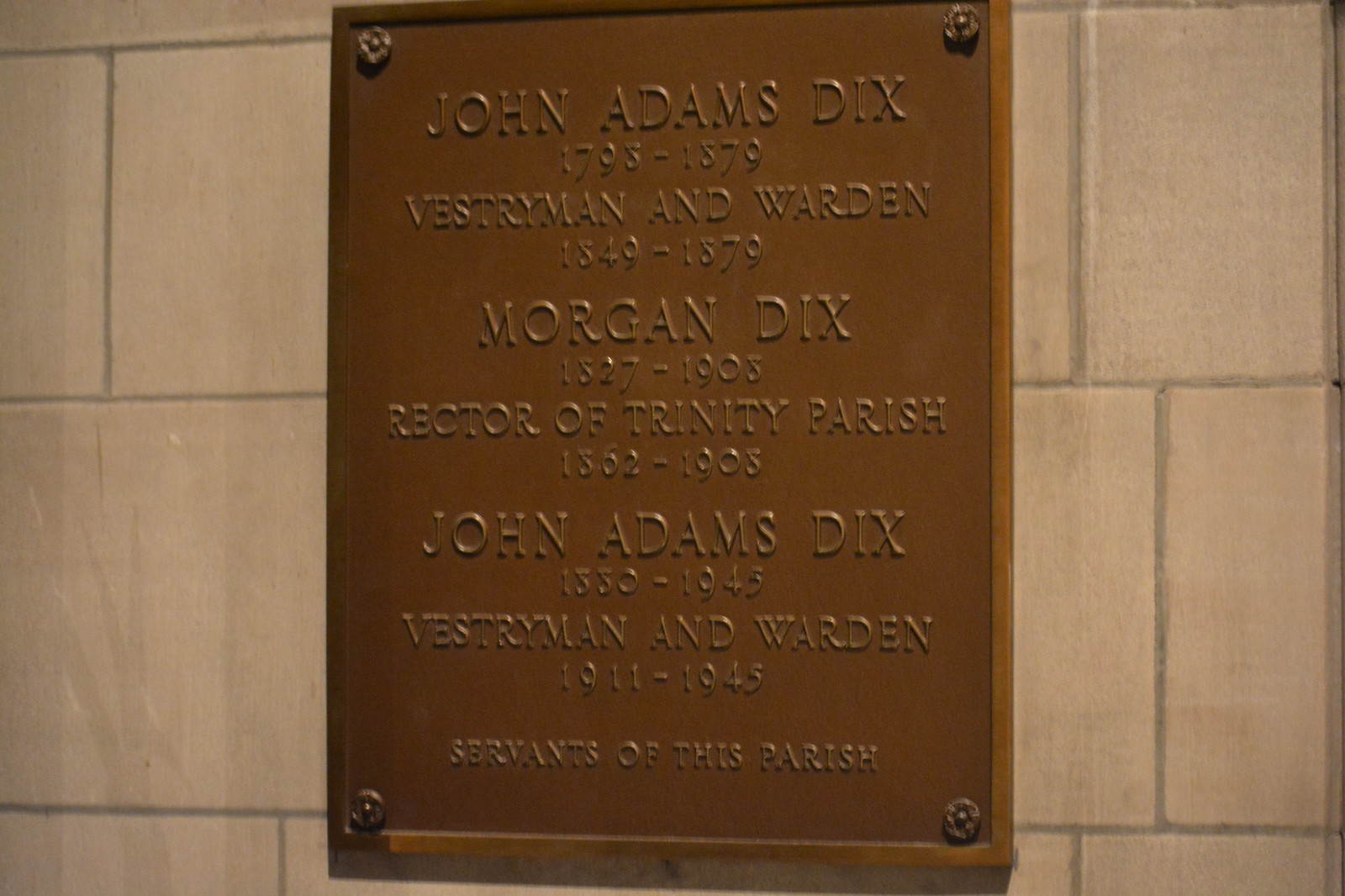This indoor photograph captures a bronze plaque affixed to an off-white tiled wall, possibly stone or marble. The plaque is secured in each corner by a floral-designed rivet or screw. The plaque commemorates three individuals likely related: John Adams Dix (1793-1879), John Adams Dix II (1850-1943), both noted as Vestryman and Warden, and Morgan Dix (1827-1903), who served as the Rector of Trinity Parish from 1862 to 1905. Each entry celebrates their roles as dedicated servants of the parish, reflecting their contributions to the church.